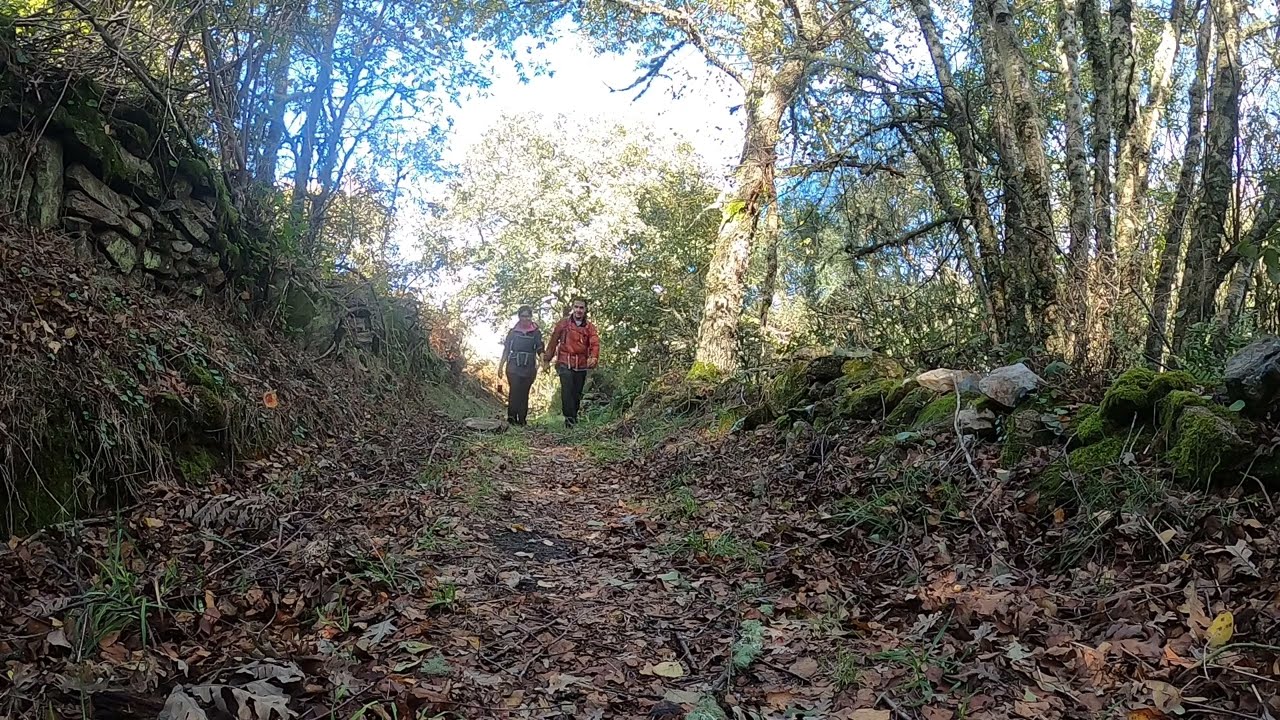In the image, a couple walks hand-in-hand along a countryside dirt path that is almost entirely obscured by an array of orange and brown leaves, twigs, and other woodland detritus. The path, sunk below the surrounding landscape, features a stone wall draped in roots and vegetation on the left, while the right side is delineated by multiple rocks. Flanking the path on both sides are towering, old, brown trees—most of which are bare with a sparse covering of green leaves.

The couple, central to the image and moving towards the viewer, consists of a woman in a black jacket and black pants on the left, and a man in a red jacket with black pants and black shoes on the right. Sunlight filters through the high-reaching branches, casting a gentle illumination over the forest scene, contributing to the serene and picturesque nature of their apparent hike or leisurely stroll. In the background, the sky peeks through the canopy with hints of blue and white clouds, adding to the overall tranquil atmosphere.